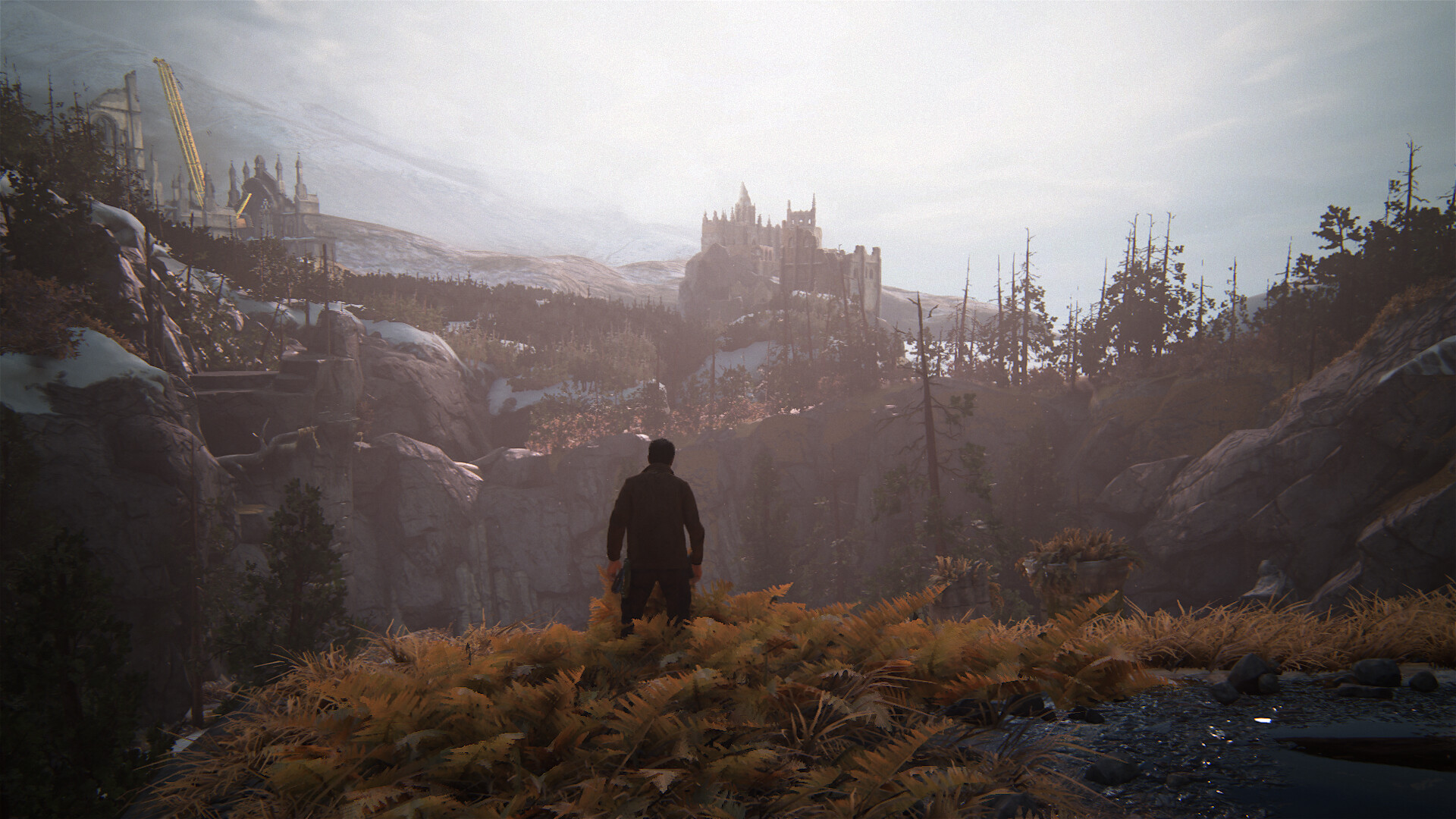The image portrays a highly detailed, photorealistic or possibly a video game still landscape, capturing a breathtaking mountainous scene reminiscent of a vast national park in the United States. At the forefront, a lone male figure, garbed in a long-sleeved robe, stands on the edge of a densely foliaged mountaintop. The foliage comprises large leaves in varying shades of green, golden brown, and yellow, reaching from his knees to his lower back. The scene suggests a transitional season such as autumn, with sunlight possibly highlighting the differing colors of the leaves.

Surrounding the figure is a rugged expanse of rolling hills and jagged peaks, extending high particularly towards the right side of the image. In the distance, a colossal castle-like structure perches on another mountaintop, while to the left, a yellow crane's boom arm angles skyward, hinting at some ongoing construction. This combination of medieval architecture and modern machinery adds a fantastical or dystopian element to the scene.

The environment below and around the cliff is speckled with scattered trees and patches of snow, particularly on opposing mountain faces, reinforcing the sense of a wild, untamed wilderness. Near the right corner, there is a small dam containing water, contributing further to the elaborate and possibly narrative-rich setting, whether from a game during a storyline moment or an illustration of a vivid, otherworldly landscape.